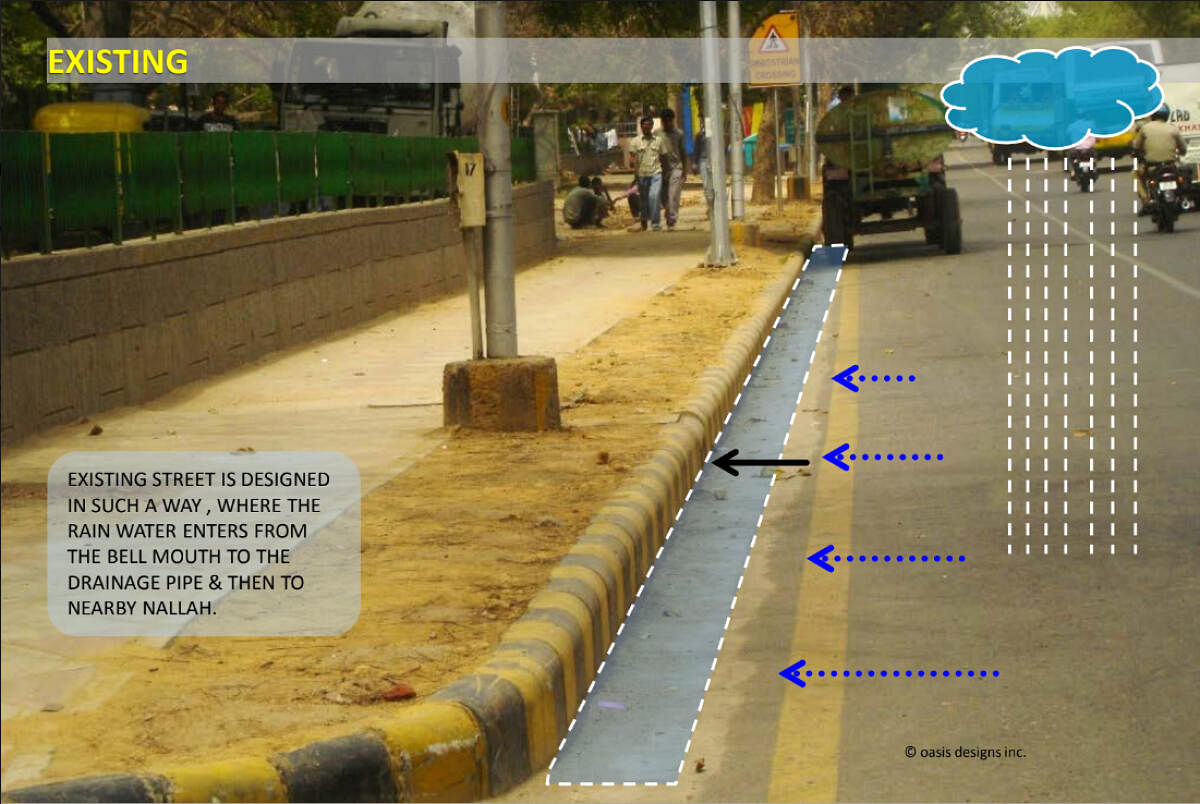The image depicts an outdoor street scene with a mix of photographic elements and overlaid graphics intended to illustrate the flow of rainwater. On the far left, a curb painted in black and yellow is visible, adjacent to a gray sidewalk with dotted white lines and blue arrows indicating the direction of water flow. The sidewalk appears in need of repair, and there is an asphalt road in the background. Above the sidewalk, in yellow capital letters, "EXISTING" is prominently displayed. A banner and several streetlights can be seen in the vicinity, along with a brick wall made of stone and some grass on the side. To the far right, a blue cloud is depicted with dotted white lines representing raindrops falling. An informative gray box on the left explains that "the existing street is designed in such a way where the rainwater enters from the bell mouth to the drainage pipe and then to nearby Nalla (N-A-L-L-A-H)." People and vehicles populate the background, enhancing the urban atmosphere of the scene.